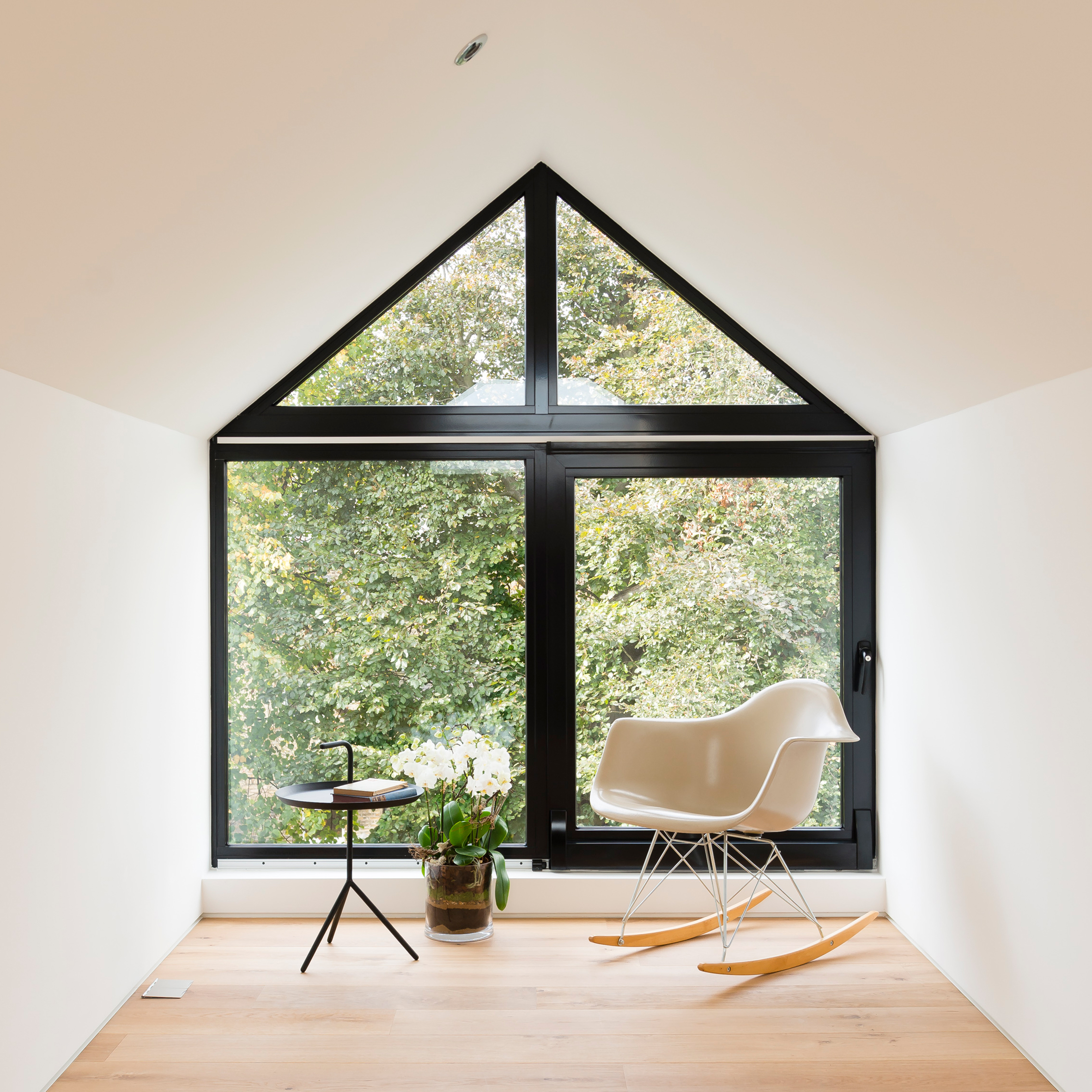In this brightly lit photograph of a simplistic room, the interior showcases a serene and minimalistic design. The room, defined by its unique architectural feature, has a large window that stretches almost the entire back wall, shaped as a rectangle topped with a triangle, resembling a classic house outline. This window allows abundant morning light to flood the room, highlighting its plain white walls and ceiling.

Against the backdrop of light brown wooden floors, the center of the room features a modern white rocking chair with metal legs and light pine rockers. Adjacent to the chair is a small, three-legged black table. Between the chair and table sits a clear glass planter with lush green leaves spilling over, enhancing the room’s tranquil ambiance. Through the expansive window, one can see the foliage of large trees and bushes, as if nature itself is invited into this intimate space. Additionally, there is a door on the right side, subtle in design, adding to the room's simplicity and functionality.